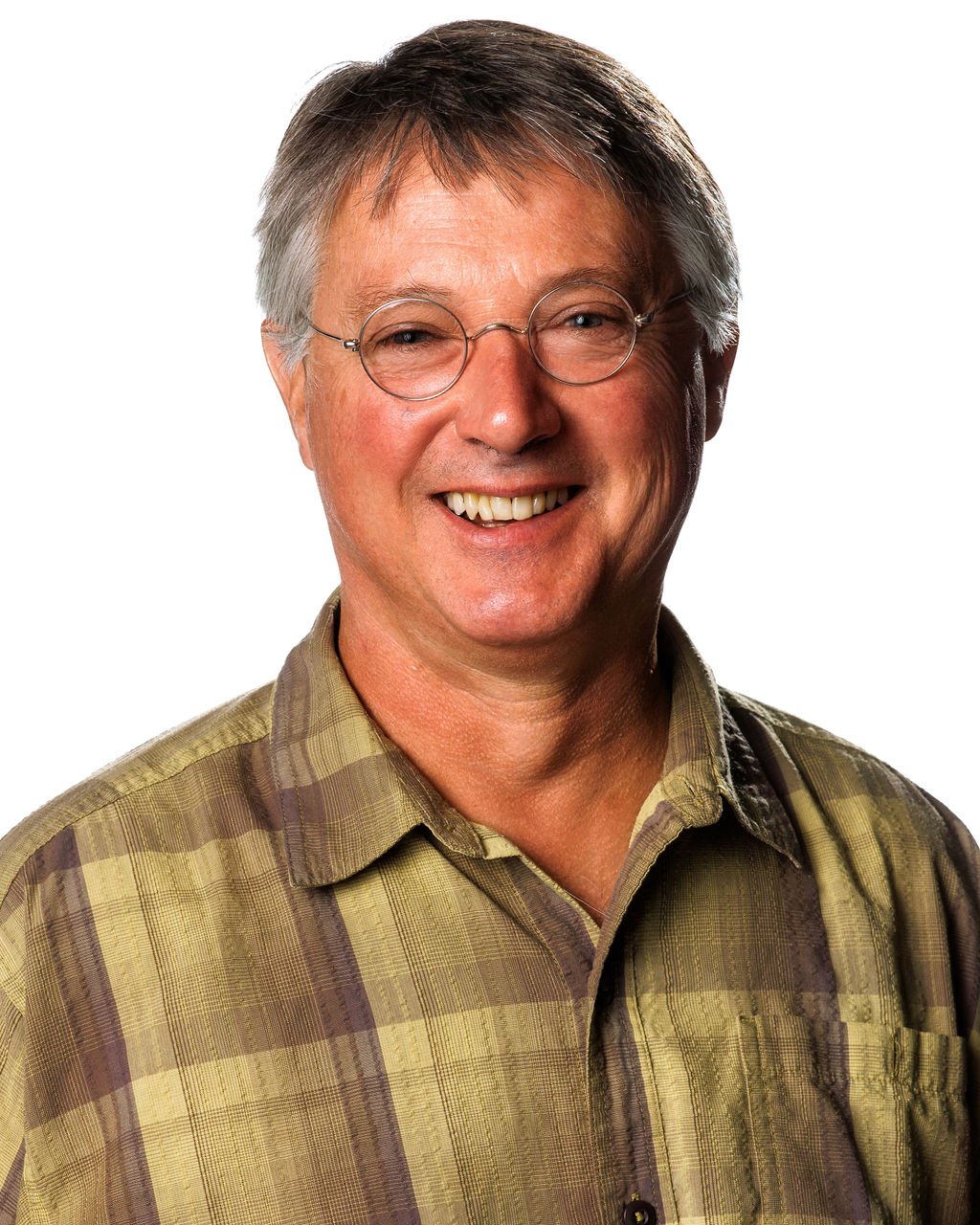The image features a middle-aged Caucasian man, likely in his mid to late 40s, with short graying hair around the sides and brown on top. He has a pleasant, wide smile that showcases his teeth, and he wears thin, silver-rimmed circular glasses reminiscent of John Denver's style. The man is clean-shaven and dressed in a button-up checkered shirt with buttoned black buttons visible near the bottom and a breast pocket on the left side (his right). The shirt is a blend of shades of green and touches of light purplish brown. The top button remains unbuttoned, revealing a relaxed demeanor. The image is vertically rectangular with a totally white background, giving no context to the setting, suggesting it was staged. The camera angle is slightly from his right, making the right side of his face slightly closer to the lens. You can see down to his mid-abdomen, and the primary colors in the image include green, yellow, skin tones, white, and silver.